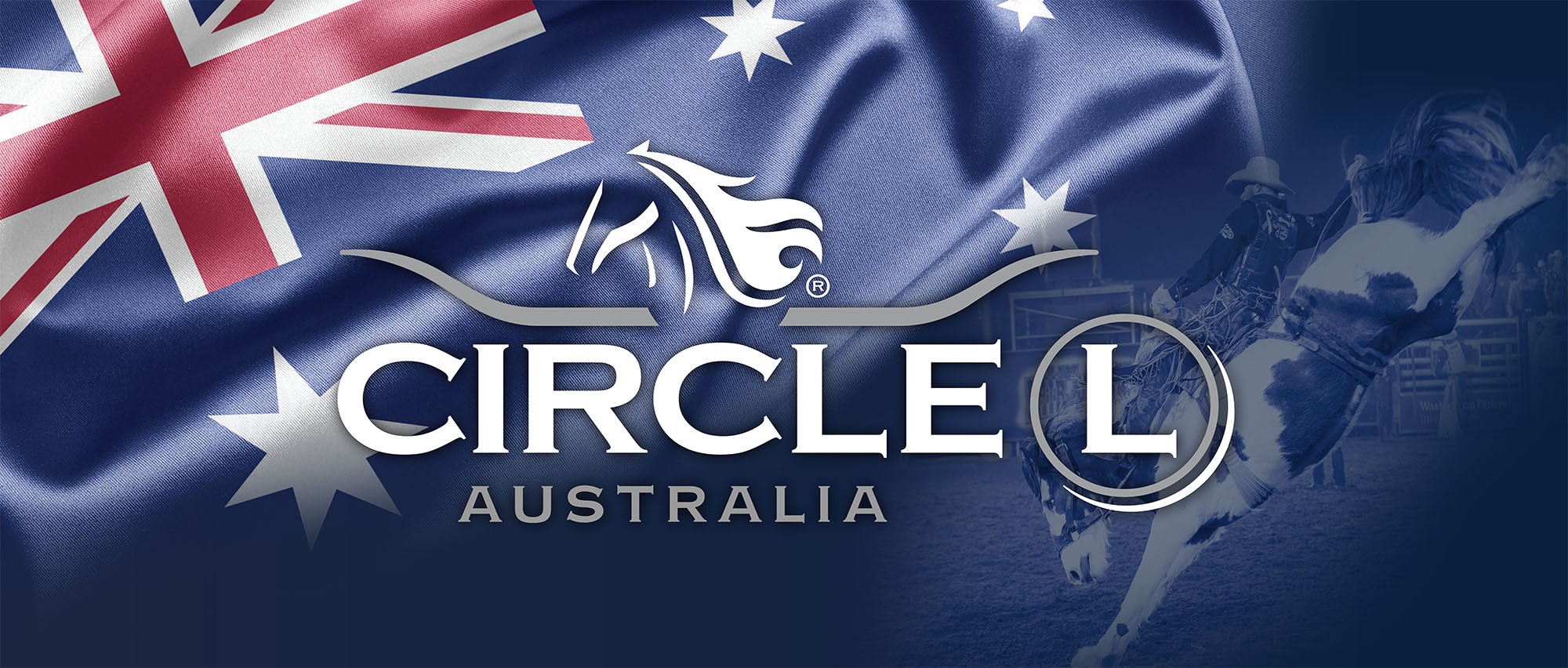The image is a widescreen horizontal rectangle featuring prominent elements against a backdrop of the Australian flag, which showcases the Union Jack in the top left corner and fades into dark blue towards the bottom right. Central to the image is a professional logo, consisting of a two-color illustration of a horse positioned above curved gray lines. Below the horse, the word "CIRCLE" is prominently displayed in large white letters. To the right of this word is a gray circle enclosing a capital white "L." Beneath "CIRCLE," in smaller gray capital letters, is the word "AUSTRALIA." Also, within the flag's background on the bottom right, there is a faint depiction of a rodeo rider on a bucking horse, accompanied by gate structures and additional figures, all rendered in dark blue hues that harmonize with the flag's colors.